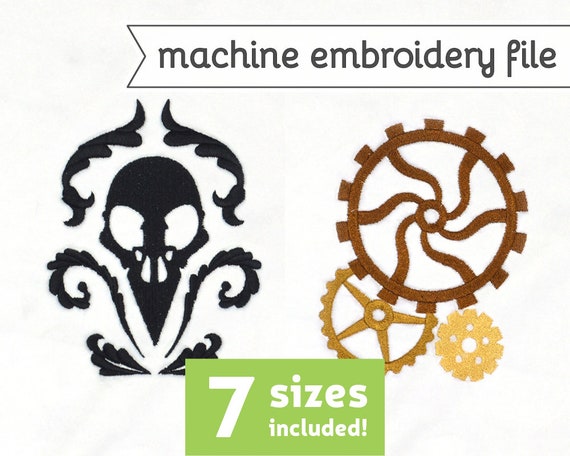The image showcases an advertisement for a machine embroidery file, prominently titled "Machine Embroidery File" in black font within a ribbon banner outlined in black, featuring a notch on the side. Below the banner, on the left, there is a detailed black skull with intricate embellishments adorning the top of its head and the neck, giving it a decorative appearance. To the right of the skull, a set of three interlocking gears is displayed: the largest gear is brown with wavy spokes, the smaller gear to the bottom left is mustard yellow with five straight spokes, and the smallest gear to the right is cream-colored with five small circles around its center. Beneath these images, a green rectangle with white text reads "Seven Sizes Included," highlighting the availability of multiple sizes for the embroidery patterns.